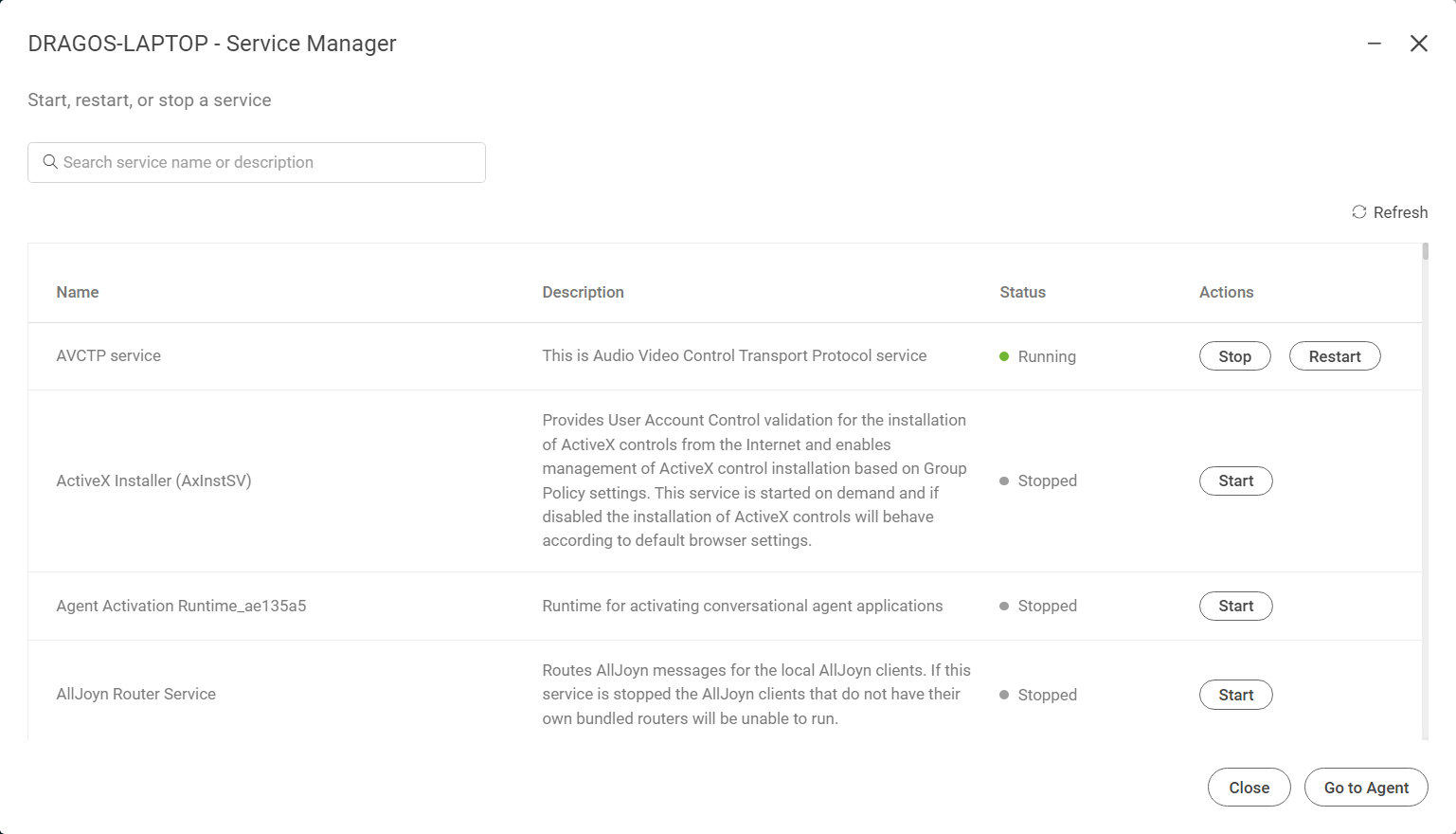This screenshot captures the laptop screen of a service management application titled "Dragos-Laptop-ServiceManager," apparent from the upper left corner. In the upper right corner, there are standard window control buttons, including a minimize button and an X button to close the application. Just beneath the title, there are three prominent buttons labeled "Start," "Restart," and "Stop Service," likely for managing various system services.

Directly below these buttons is a search bar designed for users to quickly locate specific services. To its right, there is a refresh button to update the service list view. Under this toolbar, there is a header row with four main columns titled "Name," "Description," "Status," and "Actions," laid out horizontally across the screen.

The first item listed under these columns is the "AVCTP Services." Its description reads "Audio Video Control Transport Protocol Service," indicating it deals with audio and video data transfer. The status of this service is "Running," with options to either "Stop" or "Restart" the service situated under the Actions column.

The second item in the list is the "ActiveX Installer." The description explains that this service "provides user account control validation for the installation of ActiveX controls from the internet and enables management of ActiveX controls installation based on group policy settings." Unlike the AVCTP Services, this service is currently "Stopped," and the available action is to "Start" it.

The layout, labels, and status indicators provide an organized and detailed overview of the services managed on the laptop, assisting users in service management tasks.